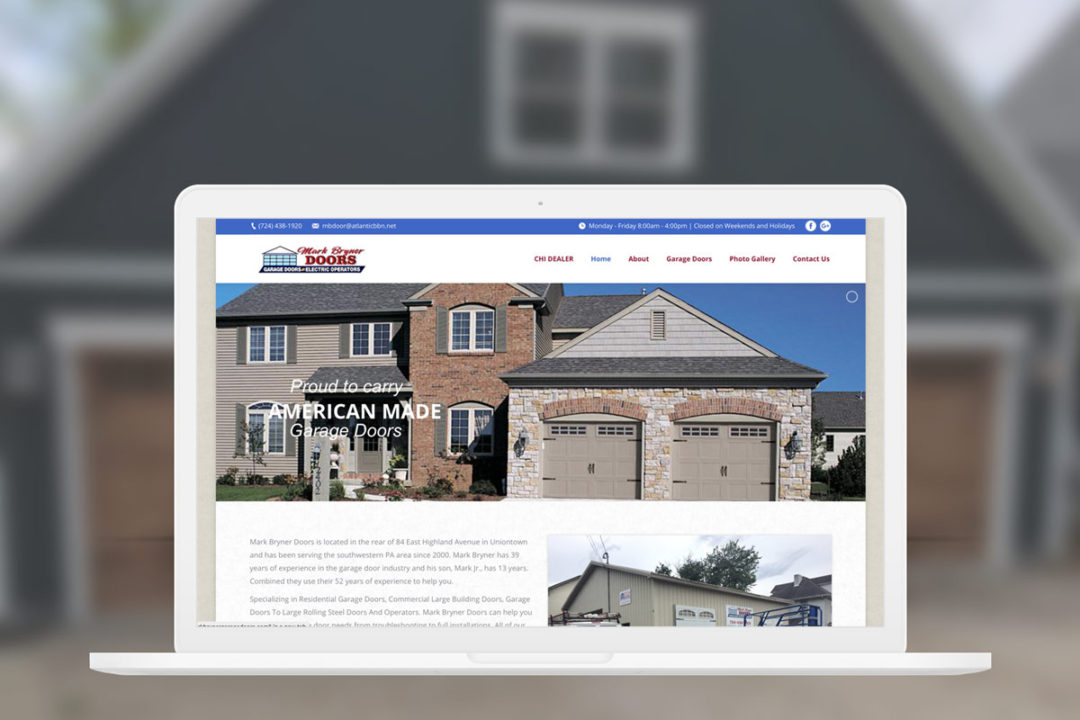This rectangular, horizontally oriented photograph features a blurred background of a house with an attached garage, displaying shades of black, tan, white, and hints of green. Superimposed over this image is a depiction of a computer screen, albeit crudely edited, showing a poorly rendered website. The website appears to be related to an electrician named Mark, with the surname possibly starting with "B," offering services related to electrical operations or garage doors. The content on this low-resolution screen includes a phone number and an email address, both displayed in white text on a blue background. A blue sidebar running vertically on the left side indicates service hours: Monday through Friday, 8 a.m. to 4 p.m., mentioning closures on weekends and holidays. There's a Facebook logo present. The header features a white band with the text "CH Dealer" and menu items—home, about, garage doors, photo gallery, contact—in red, except for "home," which is highlighted in blue. The central part of the screen shows another image of a house with an attached garage, reinforcing the theme of the website.